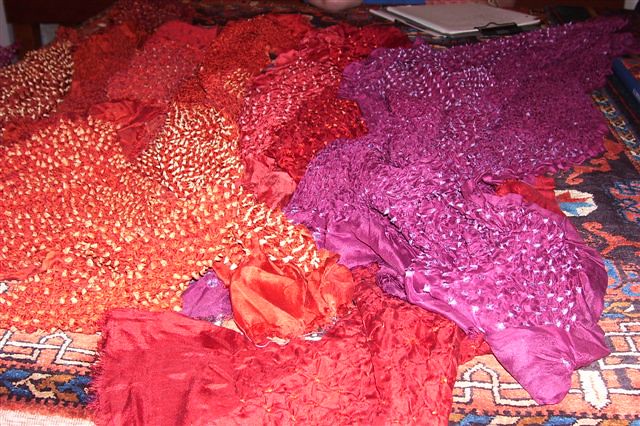This indoor close-up photograph captures a vibrant and detailed scene focused on a collection of uncut, brightly colored fabrics sprawled out on an intricate, patterned carpet. The carpet, which may resemble a Persian rug or bear an Aztec-like design, features a rich tapestry of blues, yellows, and reds in geometric patterns. Overlaid upon this are heaps of luxurious, silky fabrics in various hues such as crimson red, dark red, orange, and vivid purple, each adorned with delicate white accents or highlights that add a touch of elegance. In the background, partially visible, is a large sketch pad with a blank piece of notebook paper atop it, emphasizing the artistic setting. Additionally, a laptop can be seen in the distance, adding a modern touch to the otherwise timeless and tactile composition.